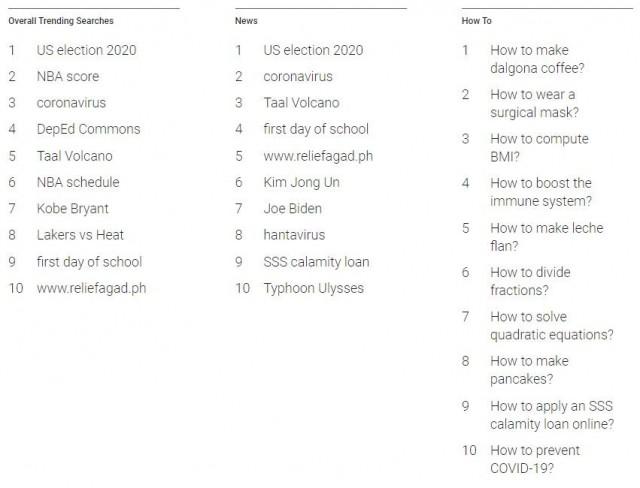The image depicts a detailed list of various search topics and their corresponding rankings. The layout is structured into multiple columns, each containing ten entries. 

- The first column is headed "Overall Train Searches" and contains: 
  1. U.S. Election 2022 
  2. MBA Score 
  3. Coronavirus 
  4. Deadbed Comments 
  5. Tall Volcano 
  6. MBA Schedule 
  7. Kobe Bryant 
  8. Lucas 468 
  9. First Day of School 
  10. www.relief.gov.ph

- The second column re-lists some of the topics under different rankings:
  1. U.S. Election 2022
  2. Coronavirus
  3. Tall Volcano
  4. First Day of School
  5. www.relief.gov.ph
  6. Kim Jong-un
  7. Joe Biden
  8. Antivirus
  9. Calamity Loan
  10. Typhoon Ulysses

- The third column is labeled "How to" and features instructional searches:
  1. How to Make Dalgona Coffee
  2. How to Wear a Surgical Mask
  3. How to Compute PMI
  4. How to Boost the Immune System
  5. How to Make Lecithin
  6. How to Divide Fractions
  7. How to Solve Quadratic Equations
  8. How to Make Pancakes
  9. How to Apply an SSS Calamity Loan Online
  10. How to Prevent COVID-19

The entire image has a white background, and each link in the columns appears in purple, indicating that they have been clicked on. This snapshot is presumably from the back end of a website or platform that tracks user search history and popular queries.